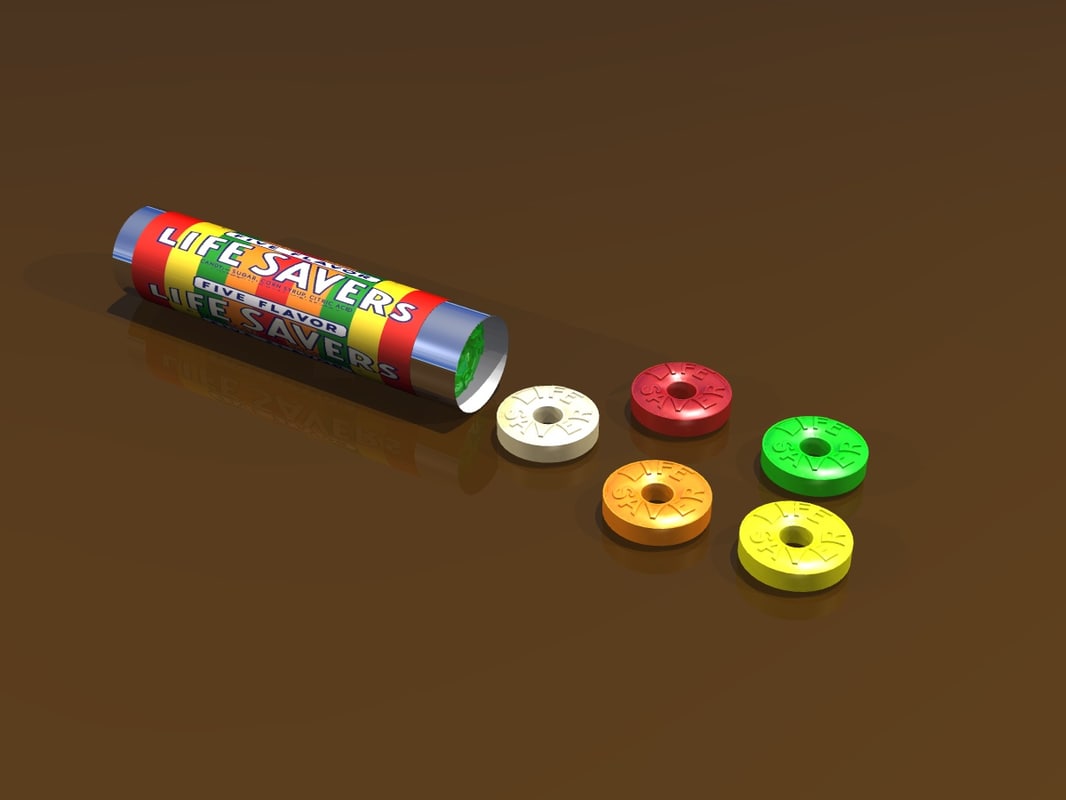The image features a pack of Lifesavers positioned diagonally on a shiny, solid dark brown background. The Lifesaver roll, located towards the left of the image, has one end open, spilling out five Lifesaver candies. These candies—white, red, orange, green, and yellow—are arranged to the right of the packaging. Each candy is circular with a hole in the center and embossed with the word "Lifesavers." The Lifesaver's packaging displays a sequence of colors: red, yellow, green, orange, and silver, with the ends of the packaging in blue. The package is clearly labeled with "Lifesavers" in white text, accompanied by the phrase "five flavors." The overall setting emphasizes the brightly colored candy against the stark brown background, making the Lifesavers stand out vividly.